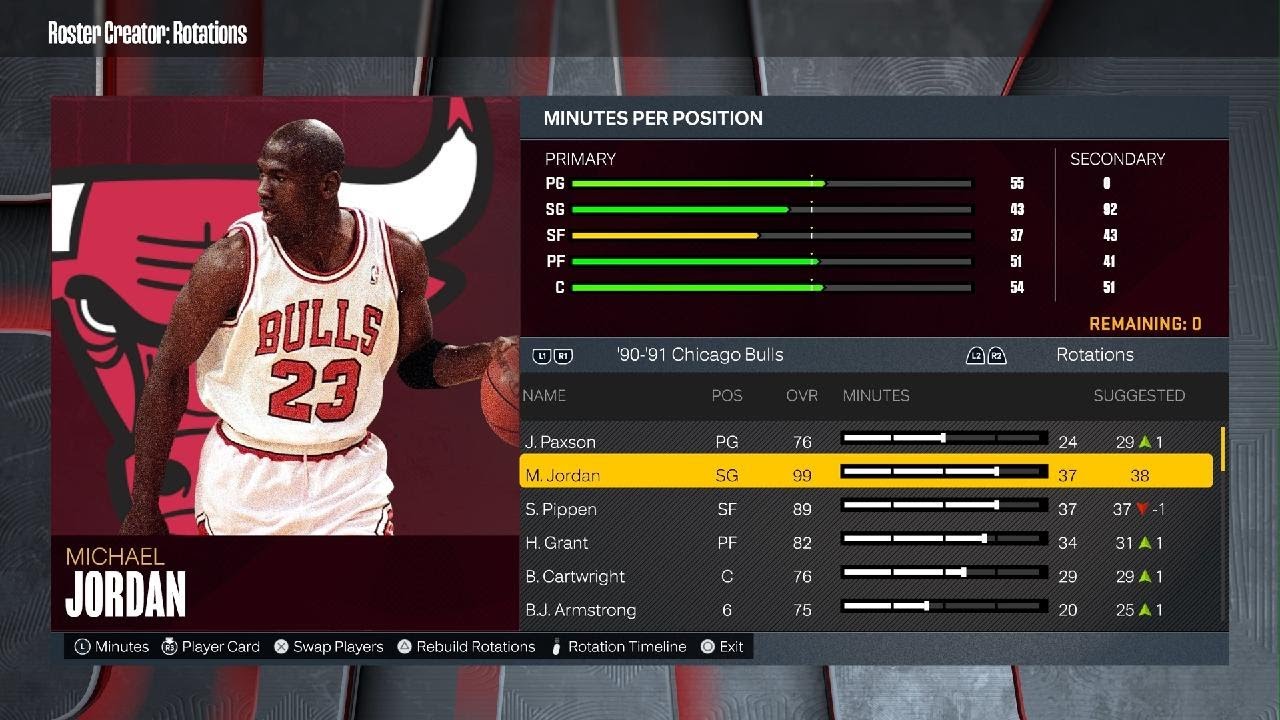The image prominently features the "Roster Created Rotations" screen with a grey and red background. On the left side, there's a detailed visual of Michael Jordan in his iconic Chicago Bulls jersey, which is predominantly red with detailed side panels. His expression is intense and focused. Jordan is holding a basketball, and behind him, a red bull with white horns is visible, complementing the Bulls' theme.

At the top of the screen, there's a section labeled "Minutes Per Position," breaking down playing time for various roles: Primary (P.G. - 55, S.G. - 43, S.F. - 37, P.F. - 51, C. - 54) and Secondary (0, running 2, 43, 41, 51) with remaining minutes at 0. Several players' details follow, including "90, 91 Chicago Bulls rotations," listing Jay Paxton as position P.G., with an overall rating (O.V.R.) of 76 minutes. Other key players like Scottie Pippen (S. Pippen), Horace Grant (H. Grant), Bill Cartwright (B. Cartwright), and B.J. Armstrong are noted with ratings of 89, 82, 76, and 75 respectively, and minute allocations such as 37, 31, 29, and 20.

Eddie Rosson's rotation tower is subtly included, suggesting Michael Jordan's minutes and player card swaps. Arrows indicating minute changes (down arrow, up arrow) for specific players are also visible. The image has grey edges with prominent red highlights, adding to the dynamic and intricate presentation of the Chicago Bulls' rotation details.